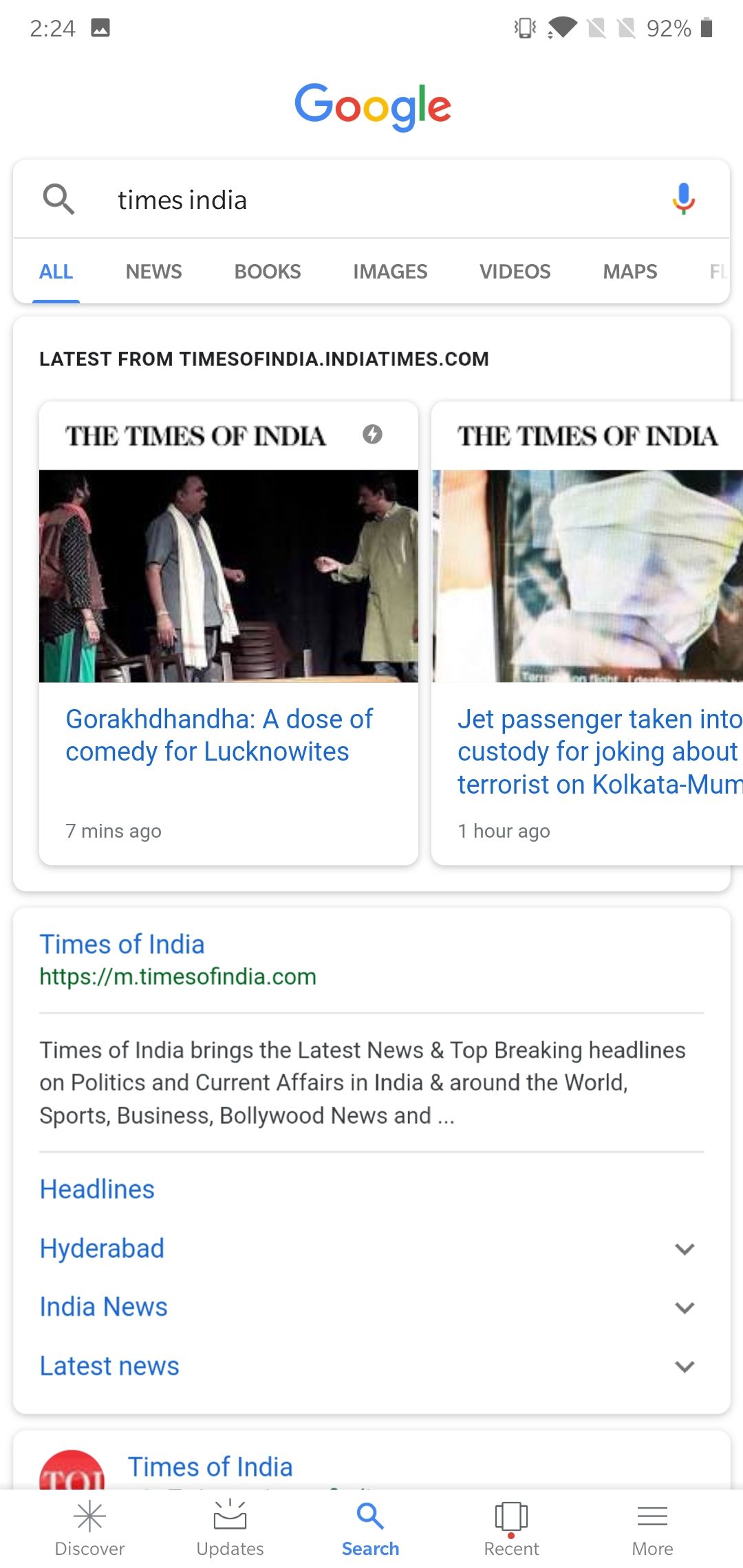A screenshot taken from an Android phone displays the results of a Google search query for "Times India." The standard Google search interface is visible at the top, featuring options like "All," "Books," "News," "Images," "Videos," and "Maps." The search results page is set against a white background.

Two search results for "Times of India" prominently appear, each marked with blue hyperlinks leading to different main pages of the Times of India website. Directly beneath the first hyperlink, the URL is shown in green, reading "https://mobile.timesofindia.com." Above the search results, the familiar Google logo is displayed. The user interface elements are standard, reflecting Google's typical search result layout.